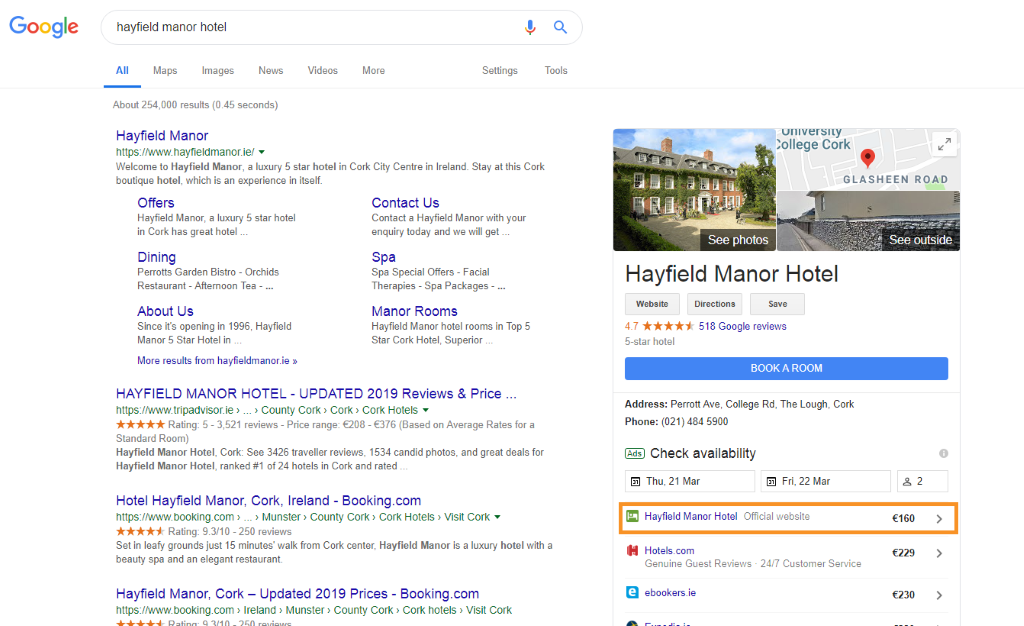A screenshot of a Google search results page for "Hayfield Manor Hotel" displays 154,000 results in 0.45 seconds. The search bar at the top contains the query "Hayfield Manor Hotel." Below, the navigation bar offers categories such as "Offers," "Dining," "About Us," "Contact Us," "Spa," and "Manor Rooms."

The primary search results feature headings like "Hayfield Manor Hotel – Updated 2019 Reviews and Price" followed by "Hotel Hayfield Manor Cork, Ireland - booking.com" and "Hayfield Manor Cork – Updated 2019 Prices – booking.com." 

To the right, there is an image of Hayfield Manor Hotel showing a tall, elegant brick building adorned with ivy. Surrounding the building are lush green trees, enhancing the picturesque ambiance.

Adjacent to the image is a map indicating the hotel's location on Glanmire Road. Below the map, options are available to view photos and snapshots of the hotel exterior, visit the hotel's website, get directions, or save the location. The hotel boasts a rating of 4.7 stars based on 518 Google reviews. Additionally, links are provided to book a room and check prices.